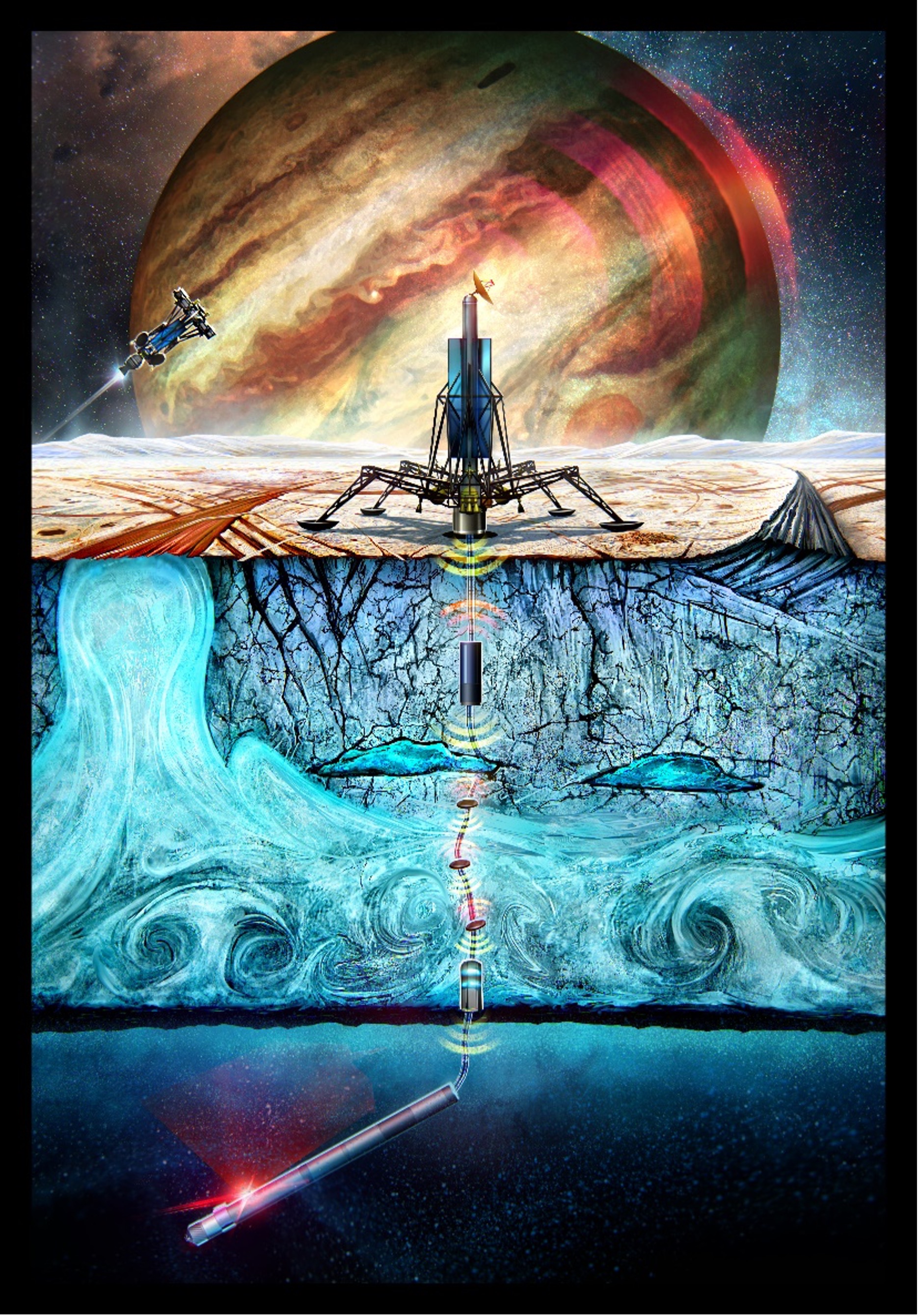This digital rendering, resembling a sci-fi comic panel, depicts an abstract scene set in space. Dominating the top third of the image is a large, gaseous planet with swirling clouds, tinged with red hues, reminiscent of Saturn but without its rings. In the foreground, a rover-like spacecraft is depicted on the planet's surface, equipped with a metal probe that drills downward through several abstract, blue wavy layers, suggesting an otherworldly representation of water. This probe is notably long, silver, and slightly glowing red at the tip, resembling a lightsaber. Adjacent to this primary rover, another smaller spacecraft hovers in the background, enhancing the sense of a multi-faceted exploration mission. The middle section of the image focuses on the drilling action, with the rover's probe piercing through different strata, extending from the rover above down through the planetary surface, emphasizing the sophisticated technological endeavor portrayed in this vivid and detailed space scene.